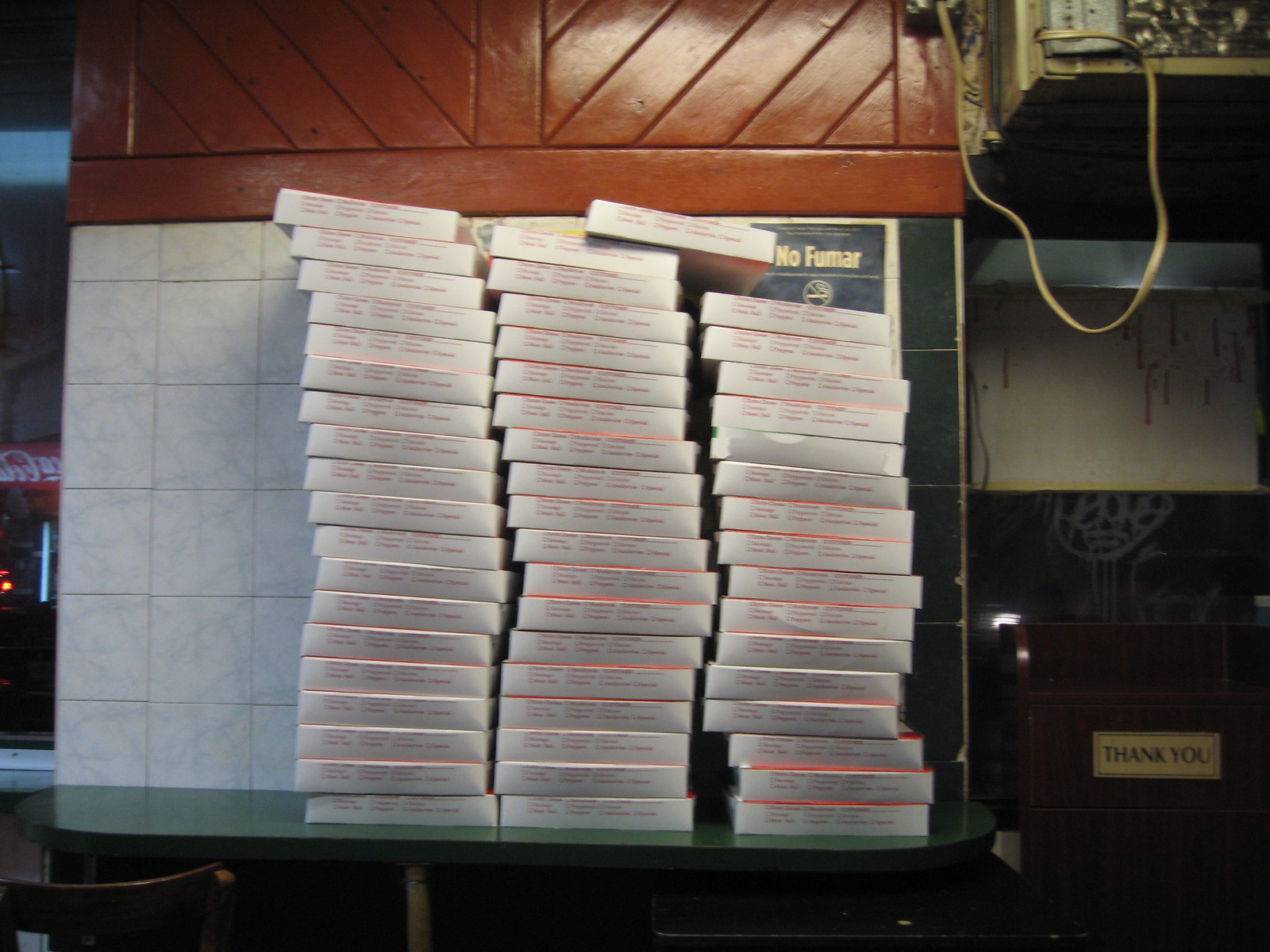This photograph captures the interior of a food-related business, likely a restaurant or pizzeria, featuring multiple stacks of boxes, possibly donut or pizza boxes, set atop a green table. The table is positioned against a tiled wall adorned with a "No Fumar" no-smoking sign, indicating the prohibition of smoking, with a crossed-out cigarette symbol. The scene includes several noteworthy elements: a brown wooden chair in front of the table, partially pulled-down large window blinds, and a yellow 'thank you' sign on a trash can to one side. Additionally, the reflection of a Coca-Cola vending machine is visible in one of the windows, which also displays some external graffiti. The background showcases red-painted boards trimming the tiled area, with cabinetry or a shelving unit above, and electrical systems visible near the "thank you" sign. The overall setting has a slightly cluttered yet functional ambiance, characteristic of a busy restaurant environment.